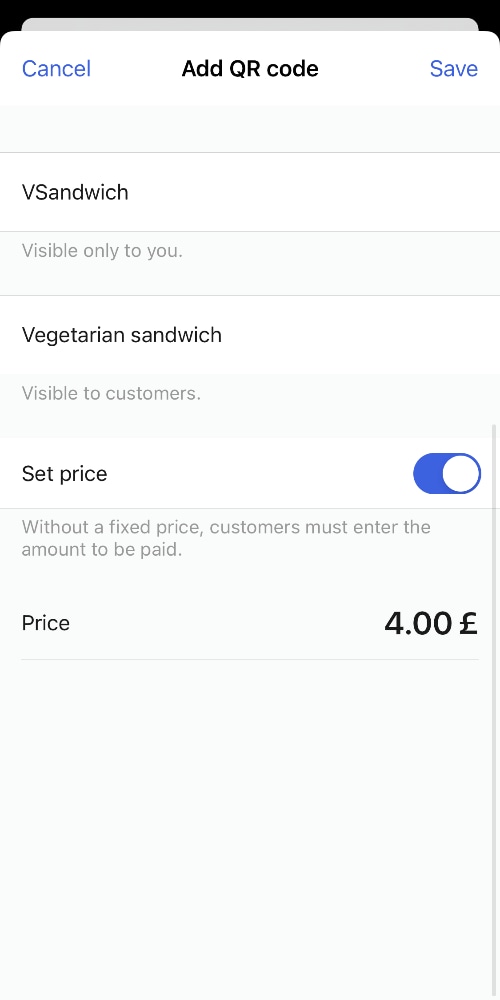This digital screenshot features a user interface for modifying a vegetarian sandwich menu item. 

- **Top Left:** A blue 'Cancel' button.
- **Middle:** A QR code.
- **Top Right:** A blue 'Save' button.
- **Text Section 1:** 
  - "VS Sandwich" 
  - Label: "Visible only to you"
- **Text Section 2:** 
  - "Vegetarian Sandwich" 
  - Label: "Visible to customers"
- **Price Configuration Section:**
  - "Set Price" option selected and highlighted in blue
  - Text: "Without a fixed price, customers must enter the amount to be paid."
- **Pricing Information:**
  - Display in black font: "Price: 4.00 [Foreign Character]"
- **Divider:** A gray line runs underneath the pricing information.